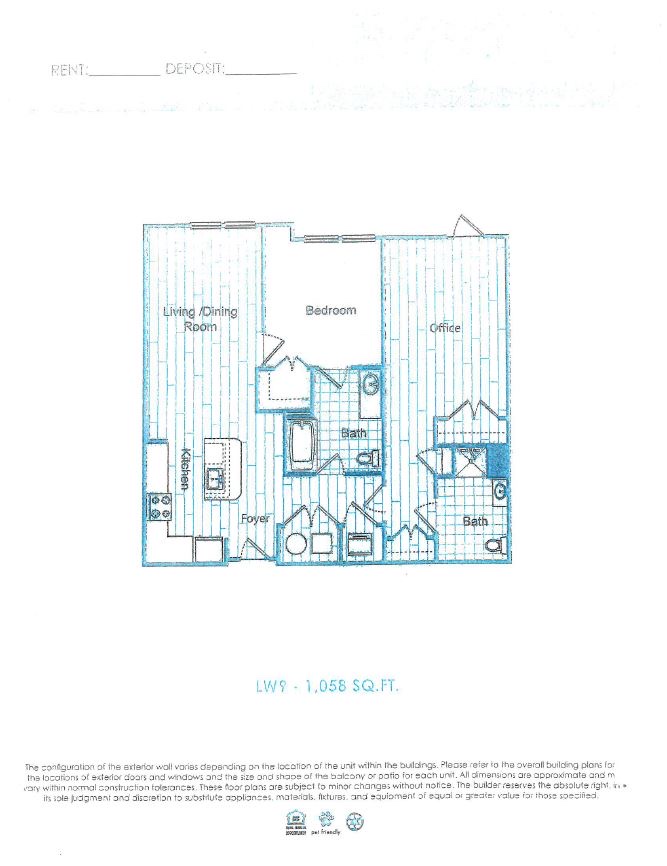**Detailed Caption of Apartment Floor Plan**

This image showcases a detailed floor plan for an apartment unit in a larger apartment complex. The layout includes multiple spaces designated for various functions, with precise labels and annotations. 

In the top-left corner of the image, there are sections labeled "Rent" and "Deposit," each with an underline to fill in the respective amounts. The unit is identified as LW9 and spans an area of 1,058 square feet. 

A disclaimer underneath the floor plan clarifies that the configuration of the exterior wall varies based on the unit's location within the building. It advises referring to the overall building plans for specific details regarding exterior doors, windows, and the size and shape of the balcony or patio. Additionally, all dimensions are approximate and may vary within normal construction tolerances. The floor plans are subject to minor changes without notice. The builder reserves the right to substitute appliances, materials, fixtures, and equipment with items of equal or greater value at their discretion.

Two icons are located near the bottom of the disclaimer, one of which is illegible, while the other indicates that the complex is pet-friendly and also supports recycling.

The floor plan lacks specific measurements but offers a general layout of the apartment's key areas. The top-left section depicts a combination living room and dining room area. Adjacent to this, in the bottom-left, is a spacious kitchen featuring an island and an entry foyer.

The central part of the floor plan includes a bedroom at the top-middle, equipped with a walk-in closet and an adjoining full bathroom containing a bathtub, sink, and toilet. To the right of the bedroom, there is a designated office space with a closet and another bathroom that includes a shower, sink, and toilet.

At the very bottom-middle of the image, there is an area likely designated as the balcony or patio, though it does not specify what could be placed in this space.

Overall, this floor plan provides a comprehensive overview of the apartment unit's layout, highlighting its various functional spaces and amenities.